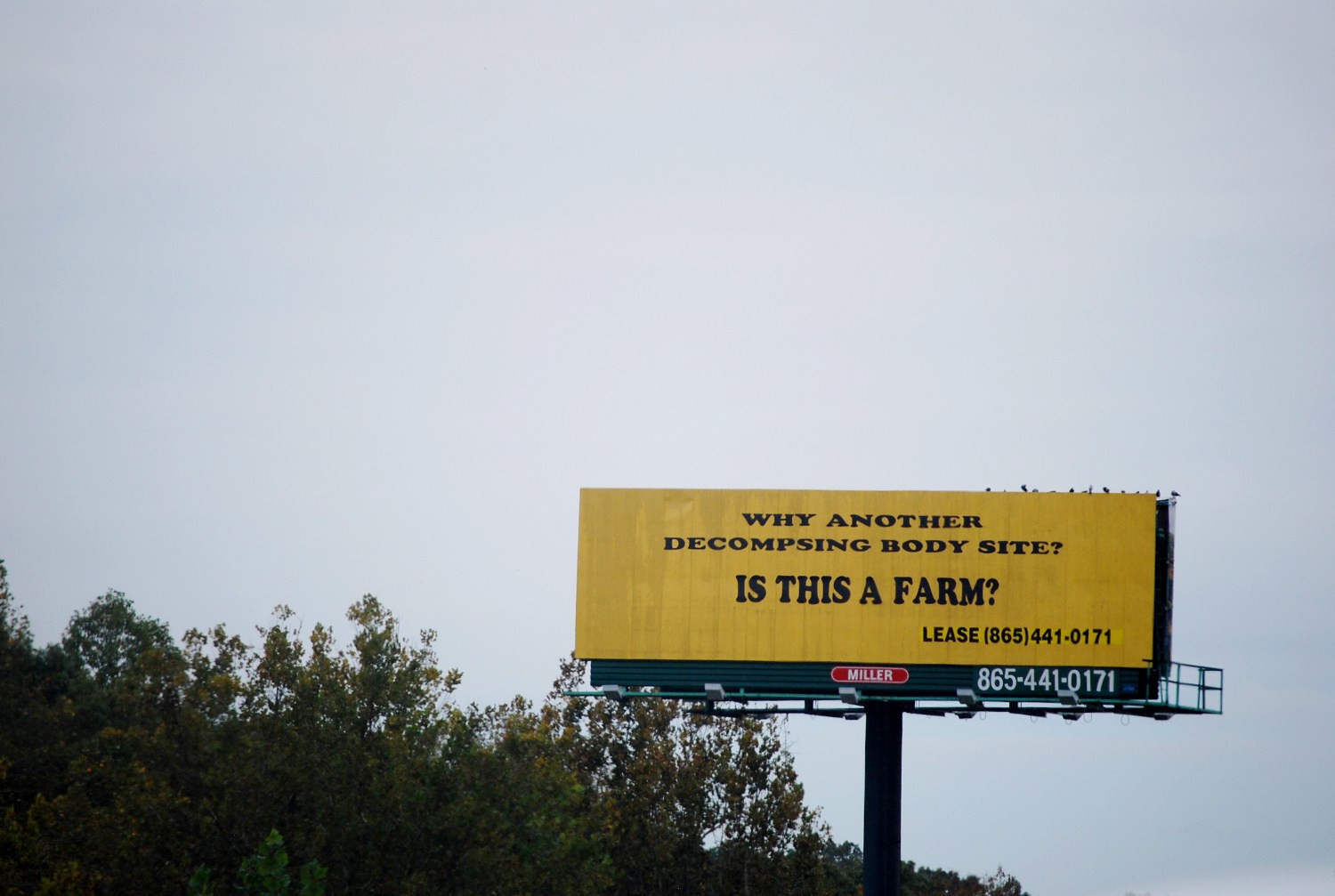A photograph captures a billboard viewed from a moderate distance, set against an overcast sky with a whitish hue, indicative of a cloudy day. The billboard itself is a long, horizontally-oriented rectangle with a mustard yellow background. Bold black letters display the provocative message: "Why another decomposing body site?" directly followed by, "Is this a farm?" Below these questions, the text "Lease" is printed, alongside a phone number: 865-441-0171. At the lower section of the billboard, an oblong red sign features the white text "Miller." The billboard is mounted on a sturdy, dark green or black metal platform, supported by a metal pole. Surrounding the billboard, both in the foreground and background, are the tops of lush trees, accentuating the juxtaposition between the natural environment and the stark advertisement.